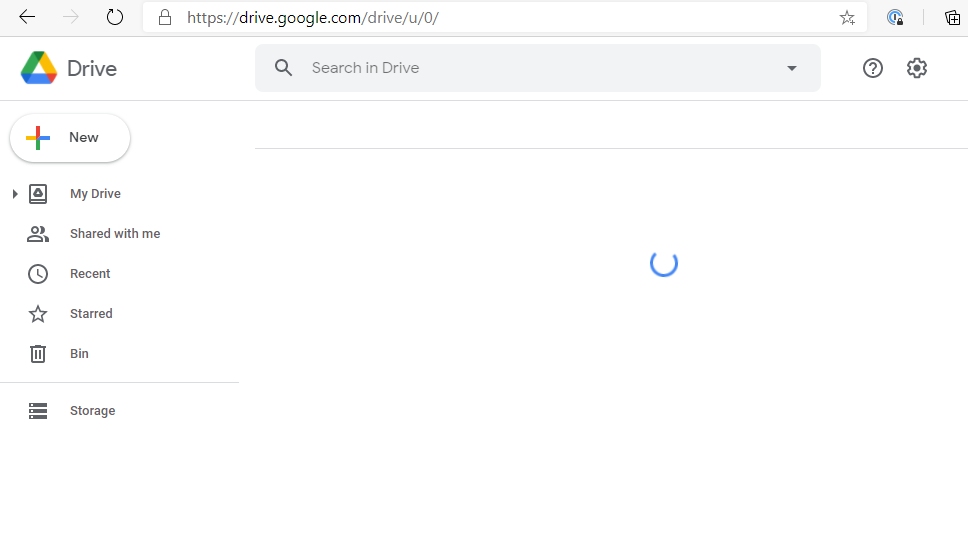A detailed screenshot of Google Drive, depicting a predominantly white interface with an emphasis on textual elements and minimal icons. At the top of the screenshot, there are two navigation arrows: one pointing left and the other right. Following these arrows is the address bar, which features a padlock icon symbolizing a secure connection, and the URL "drive.google.com." 

Directly below the address bar, aligned to the left, is the Google Drive logo next to the word "Drive." Adjacent to this is a gray search box labeled "Search in Drive," followed by a question mark icon within a circle and a gear icon, presumably for help and settings, respectively.

The left-hand column prominently displays navigation and organizational options. At the top is a colorful plus sign icon labeled "New," which appears as a highlighted button. Below this, several icons and their corresponding labels are listed vertically:
- A square icon with the label "My Drive"
- An icon depicting two people, labeled "Shared with Me"
- A clock icon next to the word "Recent"
- A star icon with the label "Starred"
- A trash can icon labeled "Bin"
- An additional icon labeled "Storage"

The majority of the page is blank, with the exception of a partial blue circle visible on the screen, adding a subtle graphical element to an otherwise text-focused layout. The overall design is clean and minimalist, emphasizing ease of navigation and use.